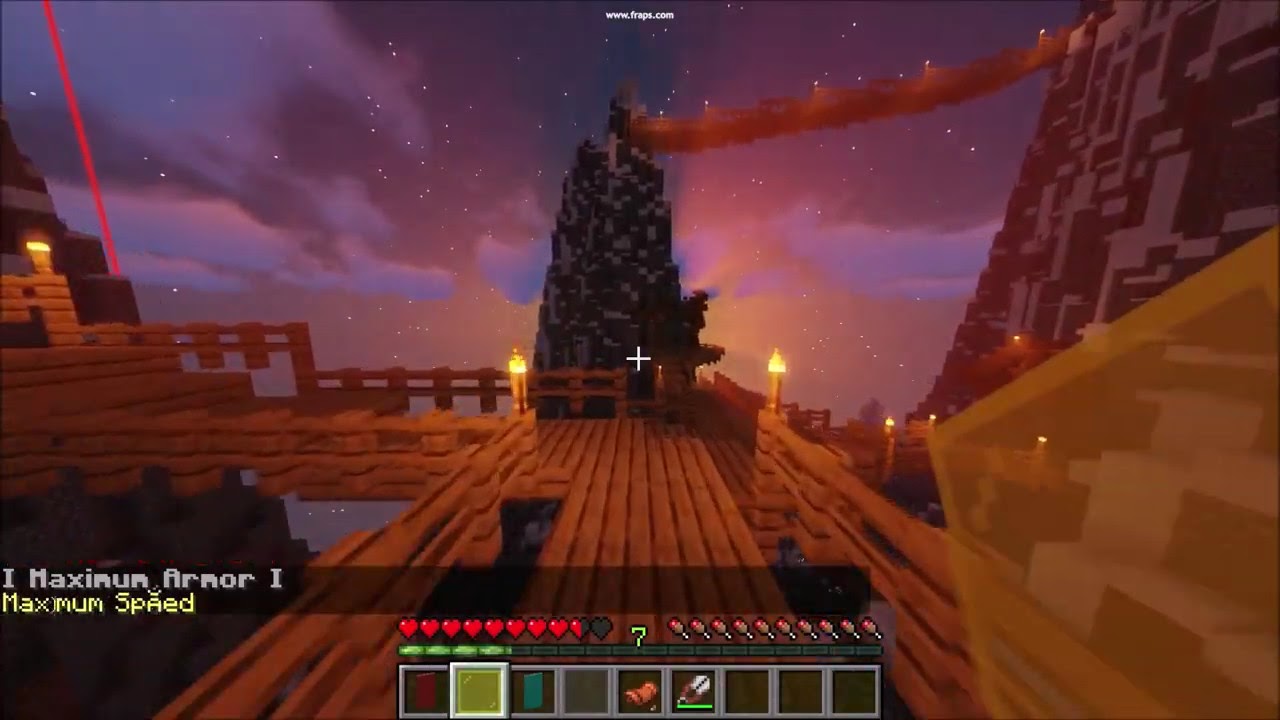This image is a detailed screenshot from a video game, showcasing a picturesque scene set against a dramatic sky blending hues of pink, gray, blue, and dark purples, reminiscent of sunset or twilight. Central to the scene is a wooden boardwalk that stretches from the foreground towards the background, where it curves to the left and slightly ascends with additional steps. This boardwalk is flanked by railings made of the same light brown wood. Scattered throughout the scene are towering granite peaks, some capped with white to suggest snow. 

On the left side of the image, white and yellowish text reads "Maximum Armor 1" and "Maximum Speed," possibly indicating the game's status indicators. The bottom of the screen features various icons, including red heart symbols signifying health, and other colorful icons that resemble lollipops and green bars. These elements are likely part of the player's HUD (heads-up display).

Amidst the game's terrain, there are additional intriguing features: a large central tree or mountain, a sky bridge, and on the right side, a tall wall with red and white symmetrical shapes, giving the impression of a complex structure. A prominent orange diamond shape also stands out on the right side, adding to the visual complexity. This rich blend of natural and constructed elements framed by a striking sky captures the immersive and fantastical environment typical of many video games.